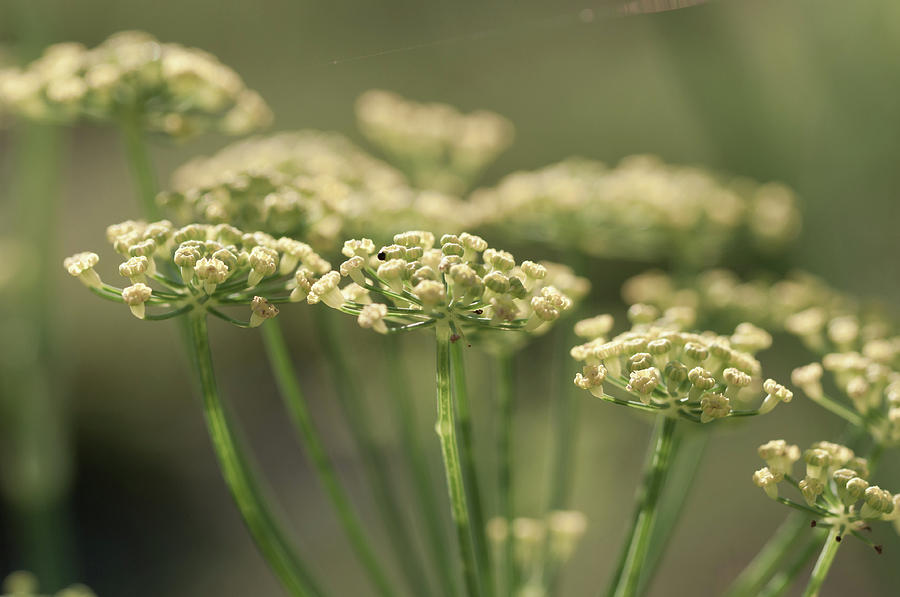This close-up photograph captures an intimate view of a cluster of Queen Anne's lace flowers, emphasizing their delicate structure. Prominently featured are four flower stalks, with long, green and light green stems that lead to tight clusters of tiny, white flower buds. These buds are shaped like small funnels, creating a lace-like effect reminiscent of baby breath. The focal flowers are sharp and clear, while the background reveals a soft focus array of additional flower stalks and heads, creating an abstract, muted blend of green and grey tones. The sunlight softly illuminates the scene, adding a gentle contrast and a hint of a spiderweb glistening at the top. The entire image exudes a natural, serene ambiance, with the detailed foreground juxtaposed against the blurry botanical backdrop.